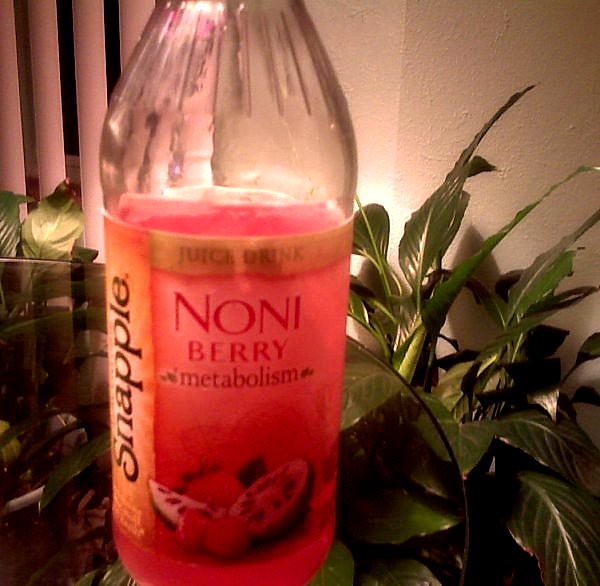This detailed color photograph features a clear glass bottle of Snapple Noni Berry Metabolism juice drink, prominently displayed on a glass table. The bottle is half-full and adorned with a pink label. At the top of the label, a gold strip with black text reads "Juice Drink." The brand name "Snapple" is printed vertically on an orange strip along the side. The main label text, "Noni Berry Metabolism," is written in a darker red against the pink background. The label also features images of various fruits, including berries, cherries, a sliced pomegranate, and possibly an apple or orange, displayed near the bottom. Behind the bottle, a green plastic artificial plant can be seen on the floor, along with long white blinds on the left side and a cream-colored wall in the background. The top left corner of the image also shows a hint of dark blinds.